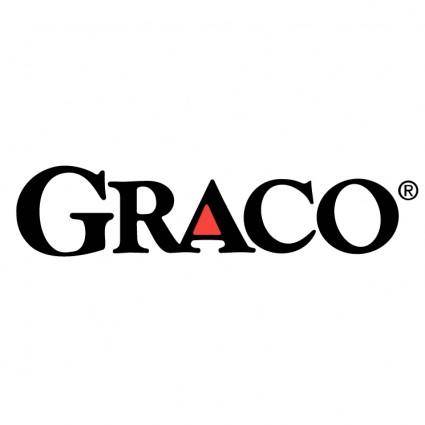The image features a simple yet iconic company logo for Graco, known for its nursery and childcare products like strollers and high chairs. The logo consists of the name "GRACO" in all capital black letters against a white background. Notably, the triangular space in the capital letter "A" is filled in red, providing the only color variation in the design. The logo includes a registered trademark symbol (®) situated to the right of the company name. Additionally, the diagonal line of the "R" flows directly into the "A," creating a merged appearance between the two letters.